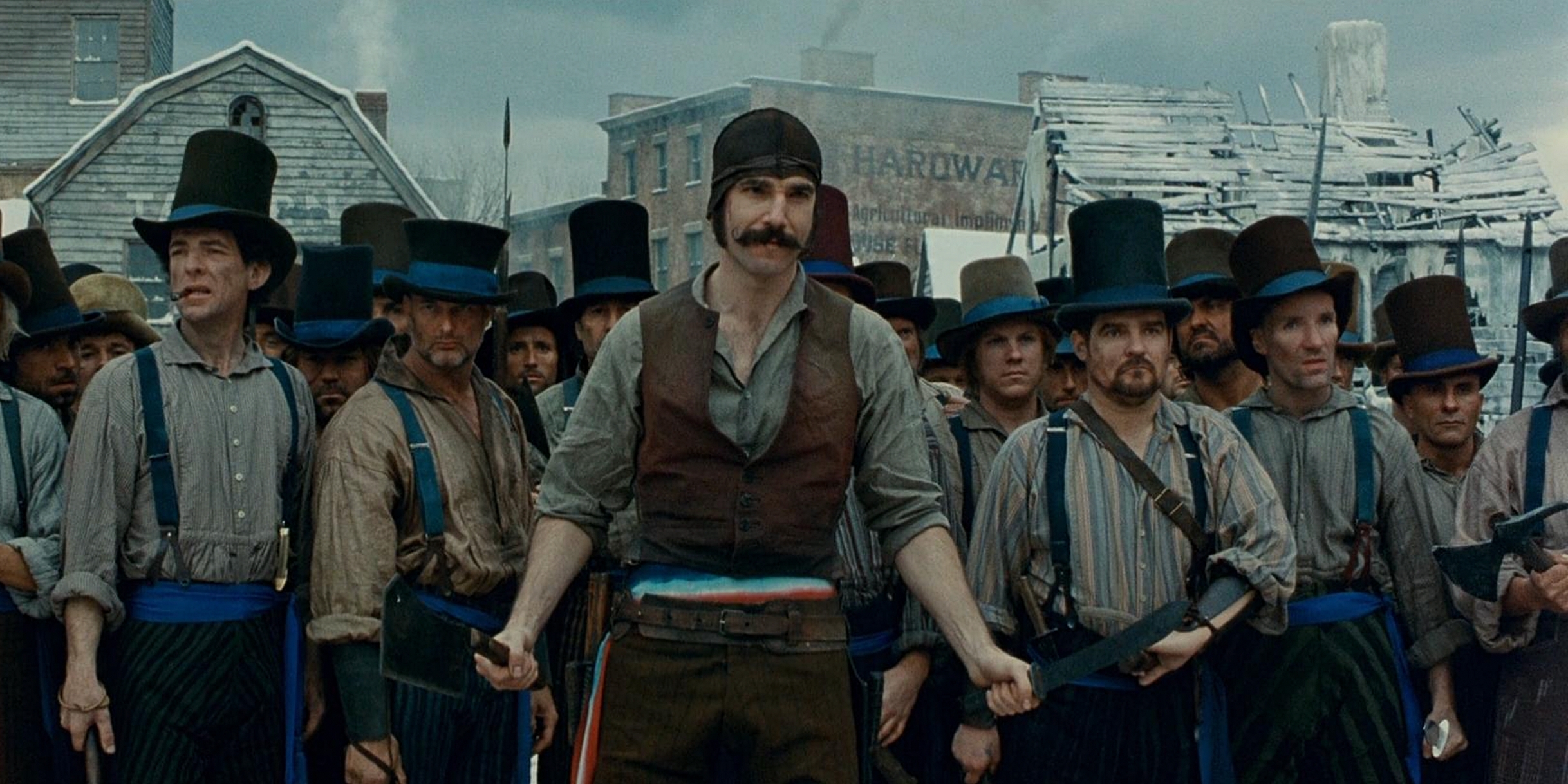The image appears to be a detailed scene from a historical movie set in the 1800s. The focal point is a group of roughly 15 Caucasian men, all of whom have a rough, tough demeanor, gathered on what looks like a dock or street, preparing for an imminent fight. Most of the men are wearing top hats adorned with blue ribbons, marking them as members of a gang, except for a central figure — a formidable man wielding large knives in both hands, and sporting a mustache and a black cap instead of a top hat. His intense gaze suggests he is ready to engage in combat, backed by his fellow gang members. The scene is set against a backdrop of decrepit buildings, one of which bears the partially visible word "Barrow." The sky is painted a stormy gray, contributing to the apocalyptic atmosphere, further accentuated by the dilapidated condition of the surrounding structures. The color palette features royal blue, black, brown, white, gray, and hints of orange, indicating a daytime setting despite the foreboding environment.